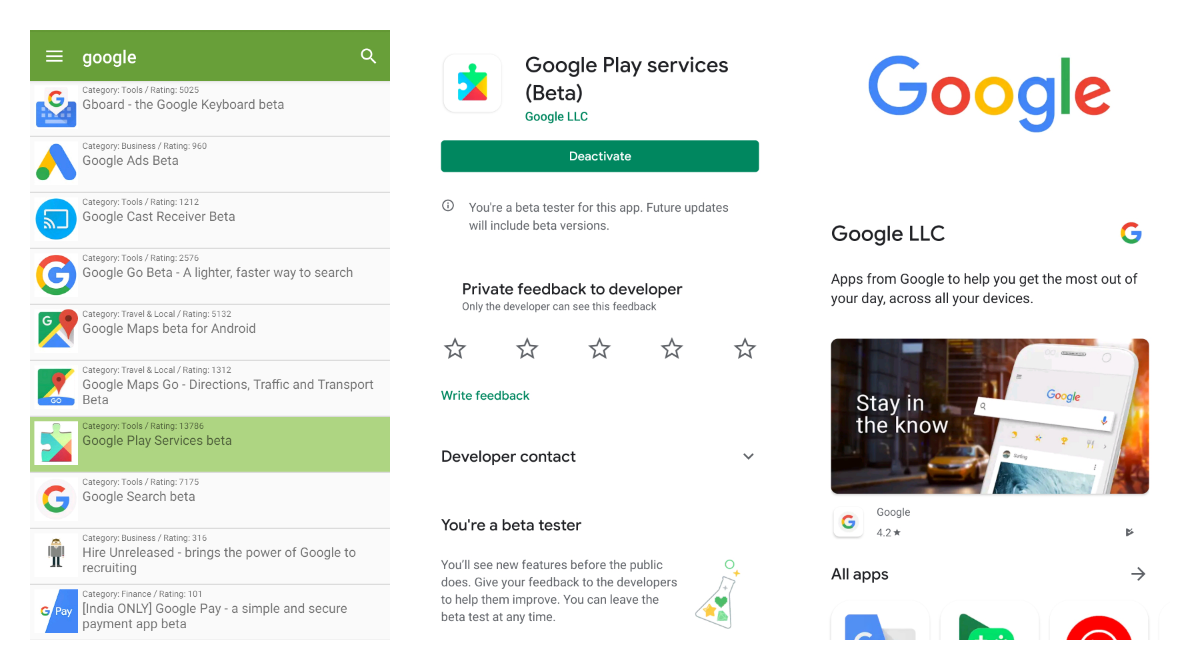In the screenshot, there are three vertically aligned pages, each seemingly captured from a cell phone. The far-right page prominently displays a large Google logo at the top. Beneath the logo, black text reads, "Google LLC, apps from Google to help you get the most out of your day across all your devices." Below this text, there is an image of a Google page open on a cell phone. On this page, it has the phrase "Stay in the know" written in white text towards the left side.

The center page is titled "Google Play Services" with a Google puzzle piece icon beside it. Directly below, there is the word "beta." A green action button labeled "Deactivate" is situated beneath this section. Accompanying this, the text indicates, "You're a beta tester for this app. Future updates will include beta versions." In bold black text, the caption "Private feedback to developer" appears, mentioning that only the developer can view this feedback. Beneath this, a five-star rating system is visible, with the subtitle "Private feedback" followed by "Developer contact." The same beta tester notice is reiterated at the bottom.